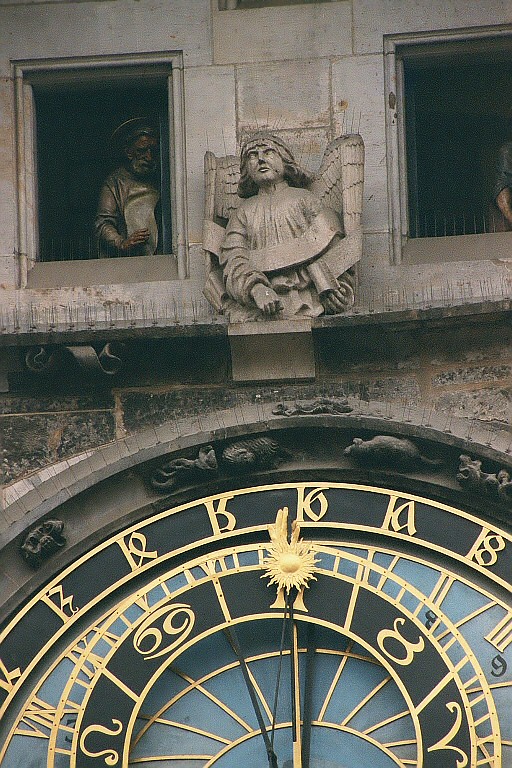This image captures the intricate astronomical clock on the facade of an ancient building, likely situated in Prague. The clock is a mesmerizing combination of artistry and craftsmanship, featuring a luxurious gold border. Its central part boasts a blue hue with a smaller black circle at the core. Surrounding this centerpiece are artistic depictions of different zodiac signs, such as Gemini, resembling the numbers 6 and 9, and Aries.

The clock's hand is uniquely designed, resembling a gold human hand, adding to the clock's elaborate detail. The areas where gold meets the background reveal a striking black contrast, enhancing the elegance of the design. Positioned above the clock is a stone figure, likely an angel. However, its somewhat intimidating appearance evokes a gargoyle-like vibe. Flanking this figure are two windows, each potentially housing another statue or a painting, though it is hard to discern due to the image's close-up focus and the relative darkness beyond the clock and its surroundings. The overall scene evokes a sense of ancient grandeur and mystique.